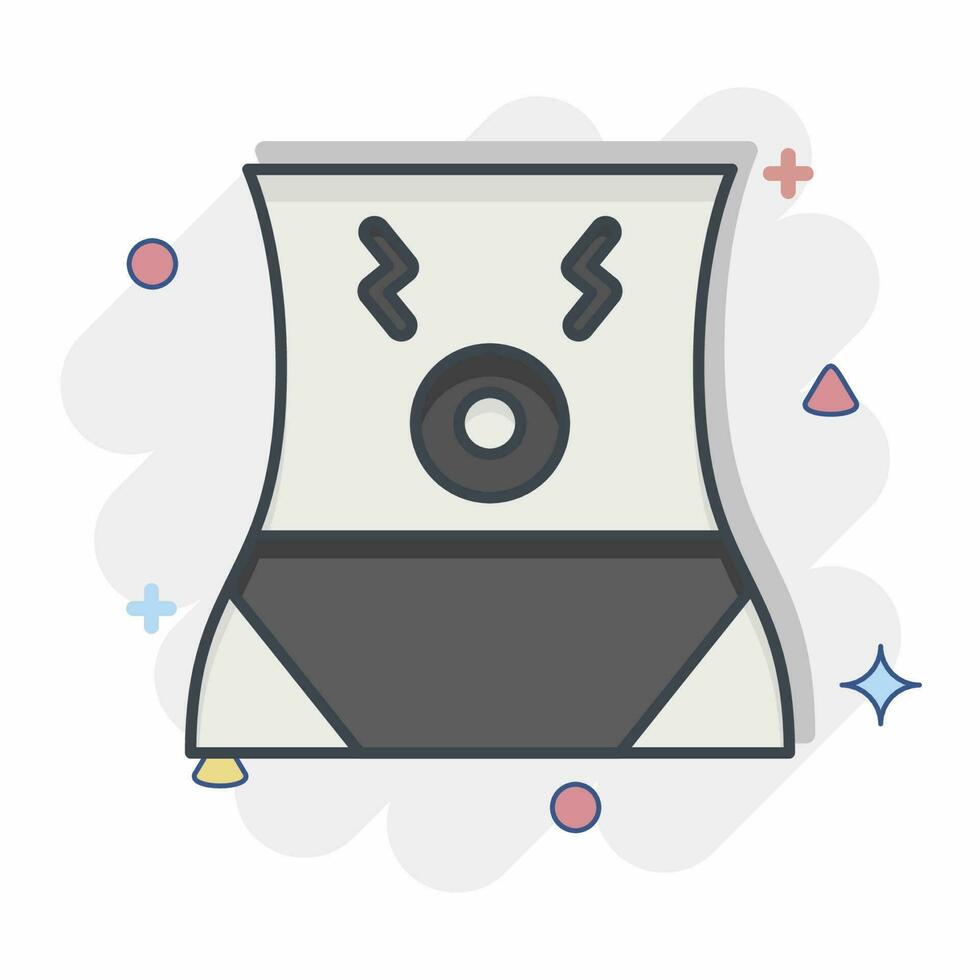The image is a digital, cartoon-style artwork primarily done in shades of black and gray on a white background with gray squiggles. It depicts the midsection of a woman's body from just under her breasts to her hips, rendered with simple, clean lines. The torso appears light gray with darker gray areas to define the shape. The belly button is illustrated as a black donut, giving the impression of an 'O' shaped nose or a shocked mouth. Above the "belly button," two Z-shaped or lightning bolt lines are positioned to resemble eyes. The figure appears to be wearing dark gray, possibly black, bikini briefs, with panty lines distinctly marked. Surrounding the torso are various small, colorful shapes, including red circles, plus signs, triangles, blue stars, yellow triangles, and blue plus signs. These shapes add a whimsical, playful touch to the otherwise monochromatic main figure.